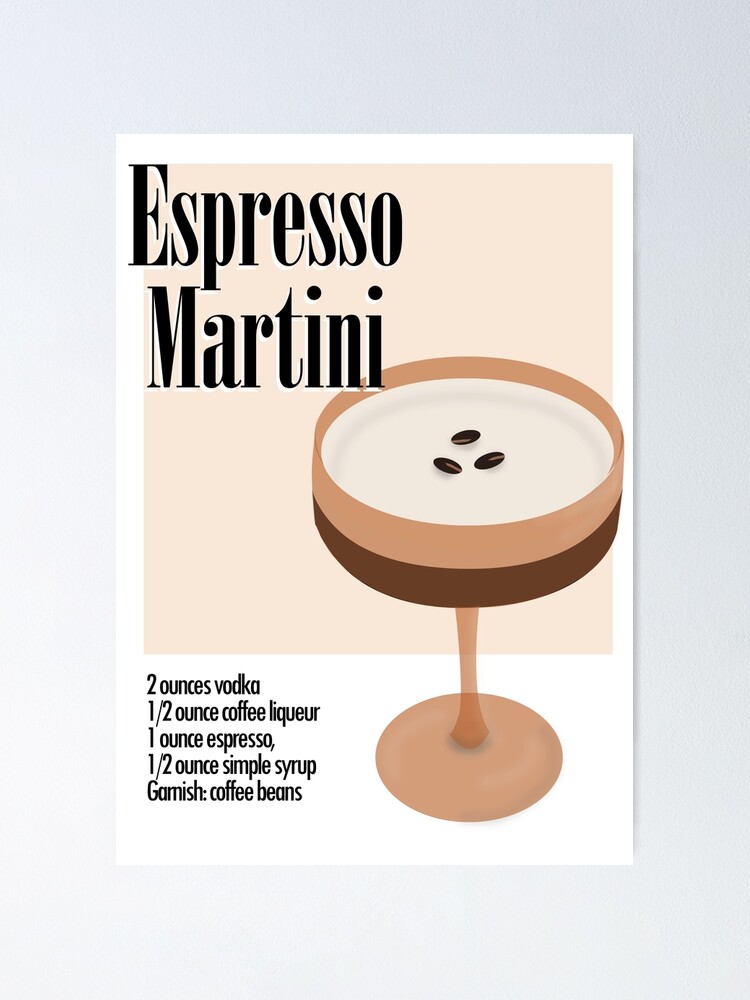The image features a minimalist poster with a clean design, set against a gray background. The main graphic, which resembles a Polaroid photo, contains a beige square with bold black letters in the top left corner reading "Espresso Martini," complemented by a subtle white drop shadow. To the right, there's a detailed drawing of an espresso martini in a shallow, circular martini glass. The drink is illustrated with a gradient from tan to dark chocolate brown, with a light khaki brown stem, and adorned with three espresso beans, arranged to resemble a face. The bottom left of the poster lists the recipe: 2 ounces of vodka, 1/2 ounce of coffee liqueur, 1 ounce of espresso, 1/2 ounce of simple syrup, and a garnish of coffee beans.